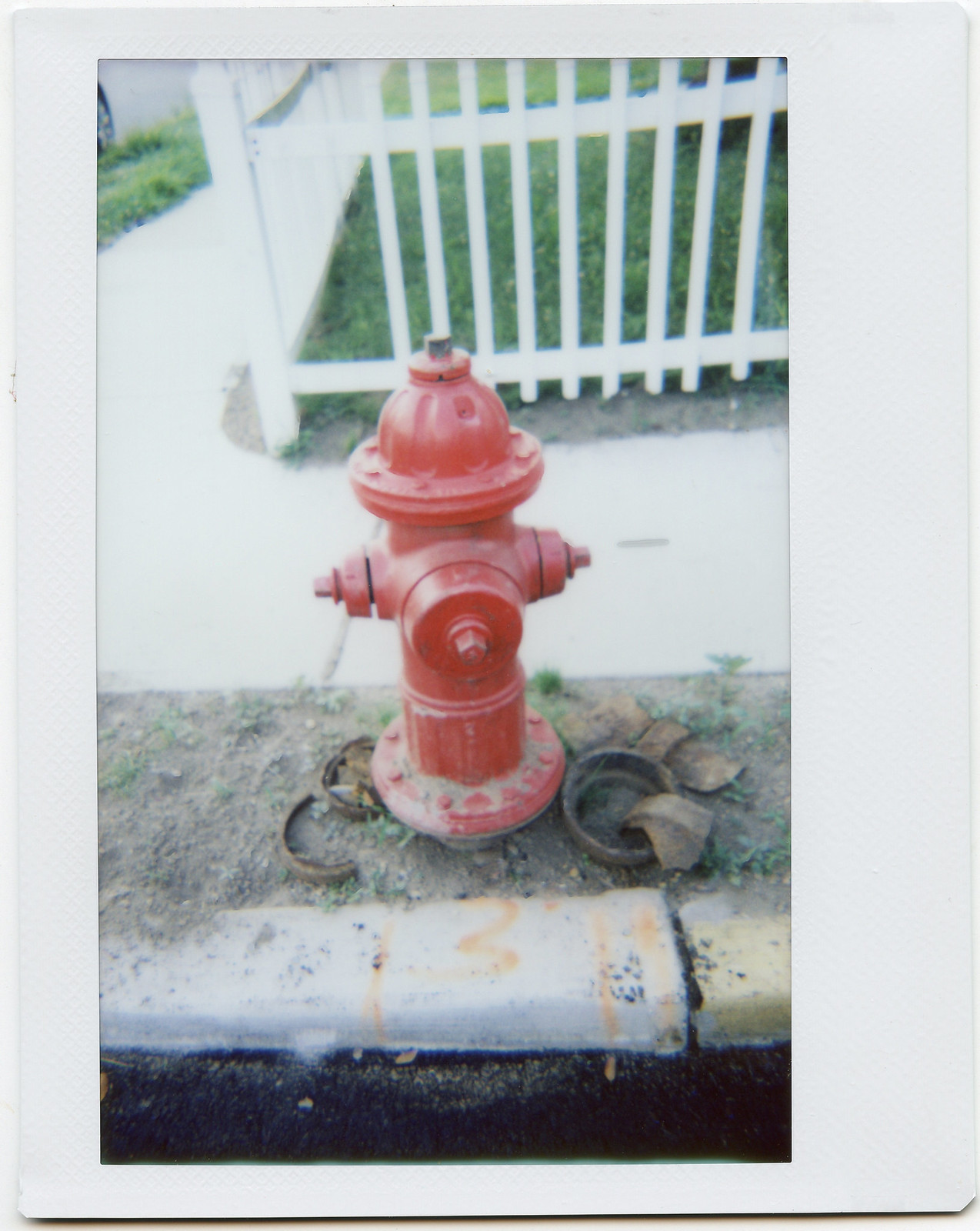This color photograph captures a prominent red fire hydrant situated on a dirt strip bordered by a black tar street and a gray cement sidewalk. The hydrant, which appears realistic, albeit somewhat toy-like, is encircled by broken metallic rings and scattered rocks. There are small sprigs of plant life around the base. The hydrant, located near a newly poured curb that curves around the location, sits in front of a white picket fence, which encloses a yard with short green grass. This fence seems to be under construction, with a few missing pickets. Some details suggest previous work on the hydrant, with markings on the curb, including orange spray-paint lines and the number three. In the upper left corner, part of a white car's wheel is faintly visible. The overall lighting makes the fence and sidewalk appear intensely white, contrasting with the darker elements in the scene.